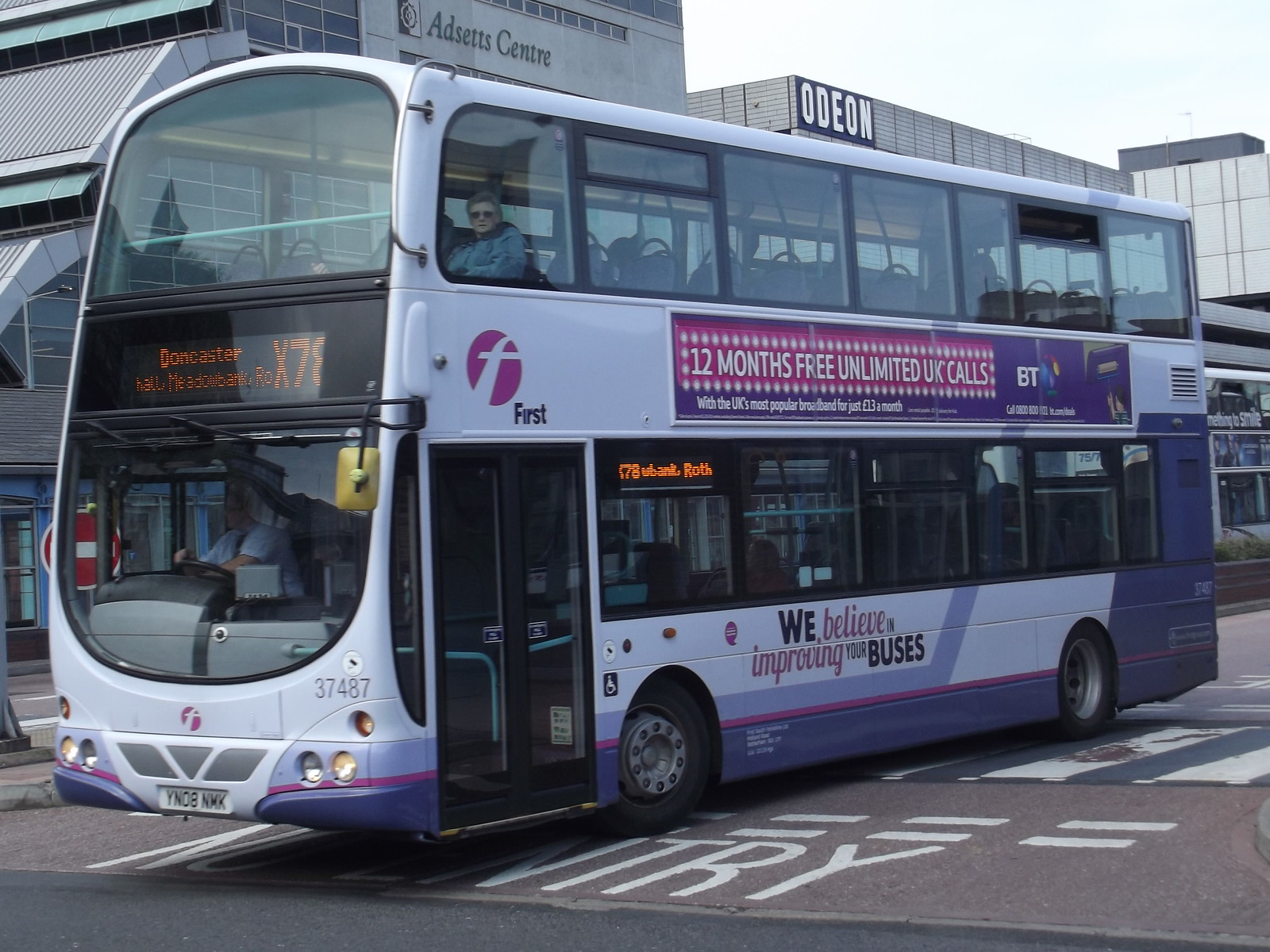The image features a modern double-decker bus primarily colored white with several purple accents. A thin purple line runs along the bottom edge from front to back, while a thicker purple stripe stretches from the front to the midpoint where it sharply ascends behind a window. On the lower level of the bus, the text "we believe in improving your buses" is clearly visible. The upper level boasts a large purple banner that states, "12 months free unlimited UK calls," with smaller text indicating it includes "UK's most popular broadband for just 13 pounds a month" by BT. The front of the bus displays LED text reading "Doncaster" with "Meadowbank" underneath, and the large designation "X78." Additionally, the bus carries the fleet number 37487 and a license plate reading YN08NMX or YN08NMK. The driver is visible through the front window. A round magenta logo featuring a white "F" is present as well. In the background, two buildings are notable: one marked "Odeon" and another labeled "ADCET Centre."